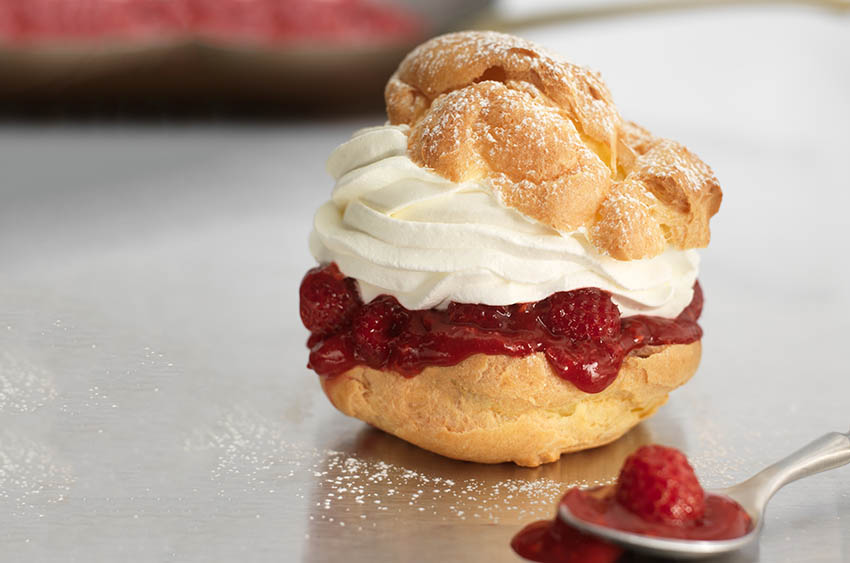The image depicts a delectable dessert composed of a biscuit cut in half, revealing a sumptuous filling of white whipped cream and juicy strawberries. The strawberries are mixed with a bit of juice, adding a vibrant splash of red that drips enticingly from the biscuit. The golden-brown biscuit is dusted with a light sprinkling of powdered sugar, enhancing its visual appeal. Adjacent to the biscuit on the stainless steel table, a silver spoon holds a single strawberry, or possibly a raspberry, along with some of its liquefied juices. The background of the image is blurred, but in the top left corner, a hint of a red and green object suggests a cut-open watermelon. The table is golden brown, complementing the dessert perfectly. Overall, the combination of textures and colors creates a visually captivating and mouthwatering scene.